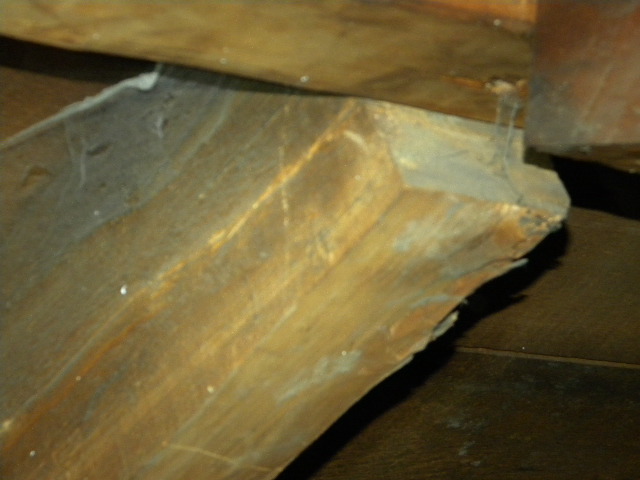This image depicts an old wooden structure, where aged beams and planks form what appears to be the framework of a building's ceiling or the underside of a roof. A significant diagonal beam, likely a 2x4, runs from the lower left corner to the upper right corner, covered in spiderwebs and a gray, dusty material that has accumulated over time. The wood exhibits signs of age, with chipped and worn-out surfaces, and areas of bluish-black discoloration suggestive of mold. Horizontal beams span the top and bottom sections of the image, creating shadows and adding to the sense of depth. The lighting highlights the detailed textures and grooves in the wood, emphasizing the structure's weathered, historic character.